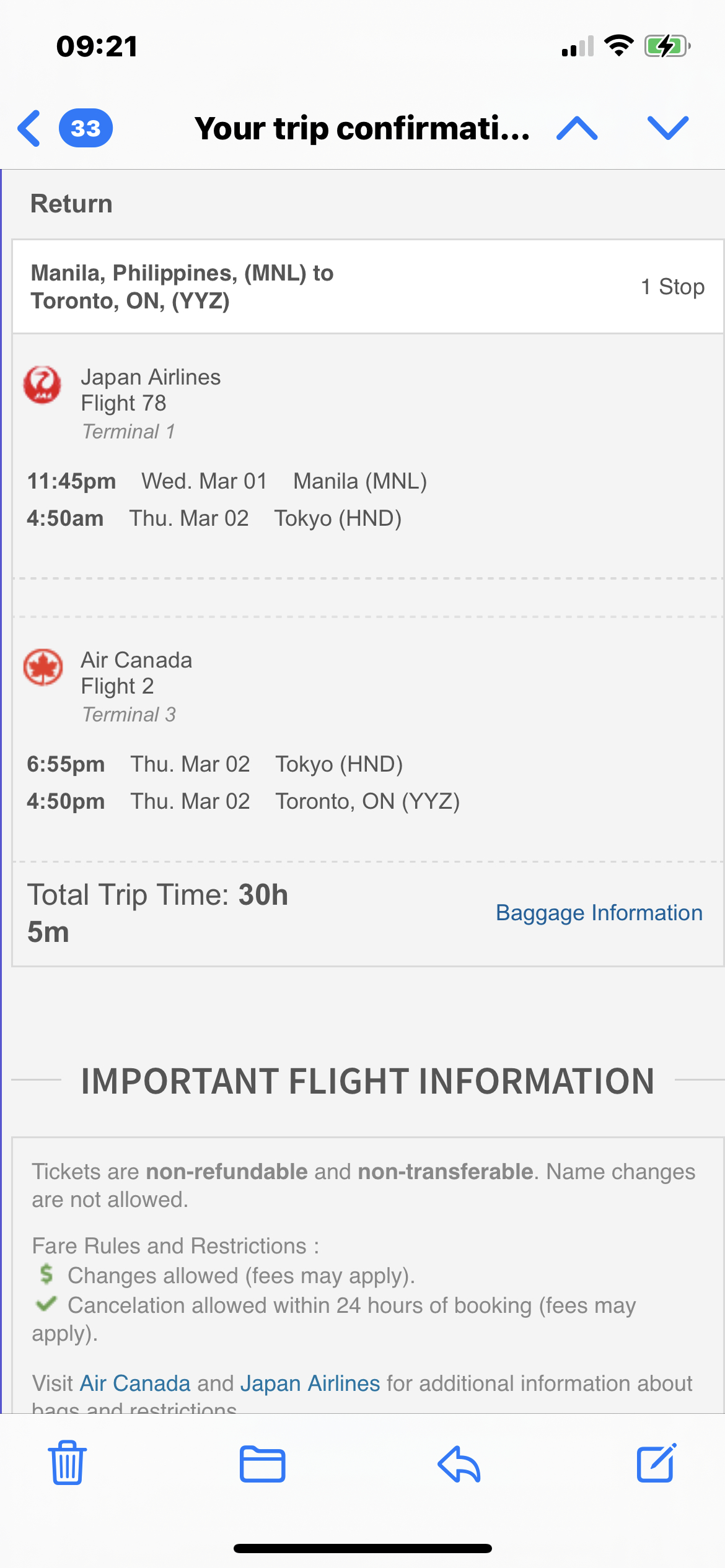Screenshot of a flight confirmation page displayed on a cell phone. At the top, the status bar shows the time as 09:21, with two signal bars indicating cellular connectivity, a Wi-Fi connection, and a nearly full, green battery icon. Below, a blue circle with the number "33" is featured next to the heading "Your Trip Confirmation."

A grey section below that reads "Return," detailing a flight itinerary from Manila, Philippines (MNL) to Toronto, ON, Canada (YYZ), with one stop. The first leg of the journey is on Japan Airlines, Flight 78, departing from Terminal 1 at 11:45 PM on Wednesday, March 1st, from Manila, and arriving at 4:50 AM on Thursday, March 2nd, in Tokyo. The second leg is on Air Canada, Flight 2, departing Tokyo at 6:55 PM on March 2nd and arriving in Toronto at 4:50 PM on the same day. The total trip duration is 30 hours and 5 minutes. 

To the right of the itinerary details, there is a section labeled "Baggage Information."

Another section titled "Important Flight Information" outlines critical travel rules: tickets are non-refundable and non-transferable, name changes are not permitted. It also mentions various fare rules, restrictions, potential fees for changes, and details on checking cancellations within 24 hours of booking. The user is directed to visit the Air Canada and Japan Airlines websites for additional information.